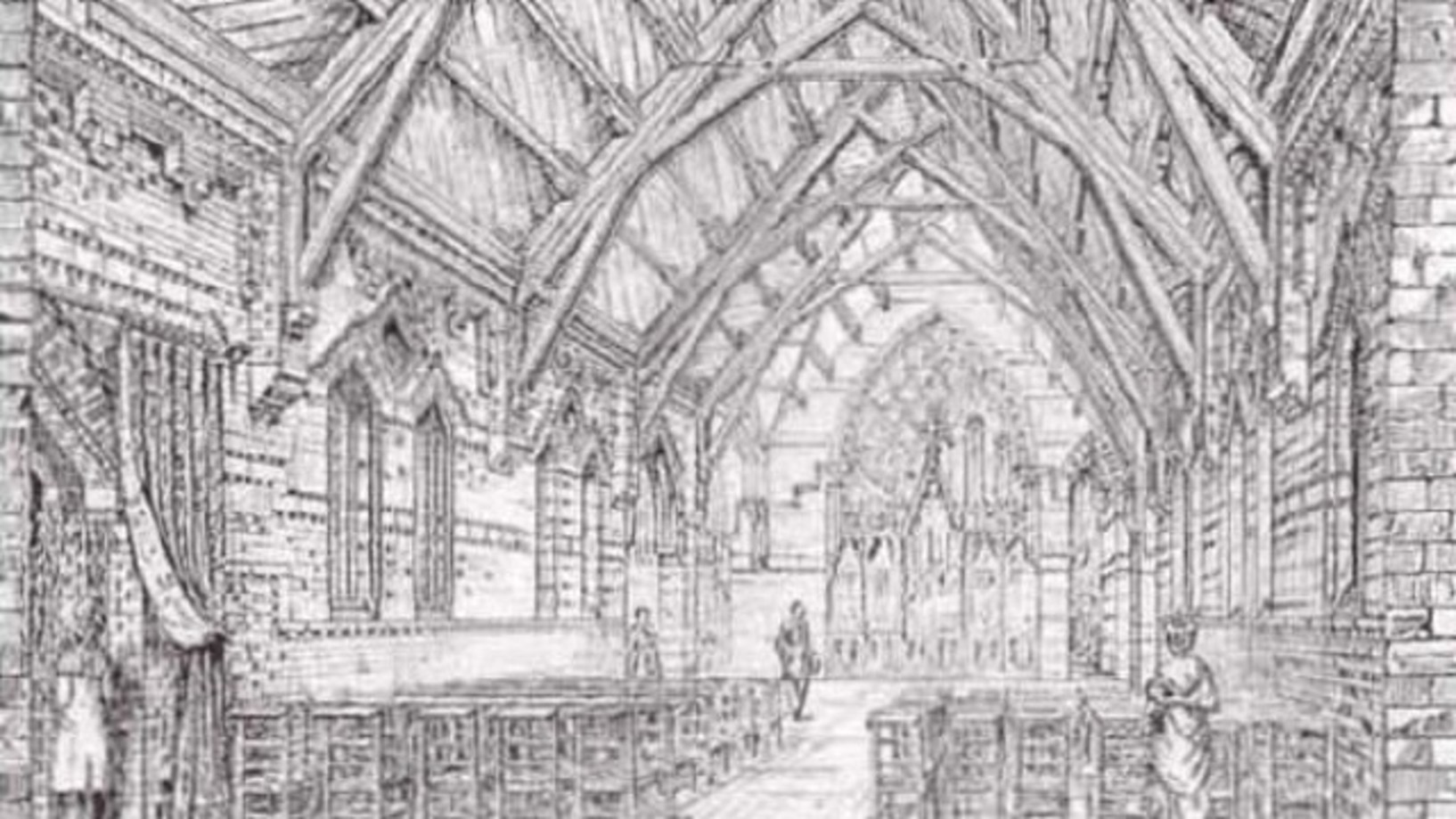This black and white, horizontally rectangular image appears to be a somewhat blurry pencil or ink illustration of the interior of a medieval church. The church's stone walls feature several large stained glass windows, accompanied by banners and other hanging cloth items. The scene is dominated by a high, vaulted ceiling with exposed wooden beams and slats. Down the center aisle, which divides chairs uniformly lined on either side, stands an altar in the far back wall, resembling a large cathedral window. The illustration also includes faint images of people; notably, to the lower left is a female figure in a light dress viewed from behind, while to the lower right another female figure, dressed in a Victorian-style long dress and bonnet, can be seen. Although details are not very clear due to the blurriness, the orderly arrangement of chairs and the overall architectural details are distinctly visible.